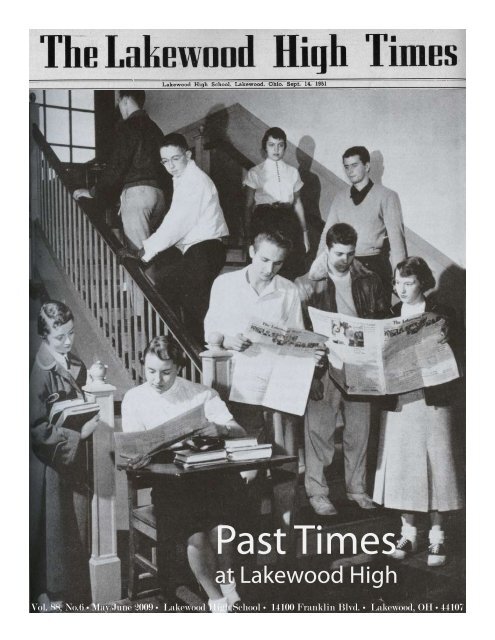This is a black and white magazine cover titled "The Lakewood High Times" at the top. The bottom of the cover features the caption "Past Times at Lakewood High" along with the address 14100 Franklin Boulevard, Lakewood, Ohio 44107 and the publication details: Volume 88, Number 6, May-June 2009. The image depicts a group of teenagers in 1950s attire, including poodle skirts and long coats, gathered on a school stairway. Several students are intently reading a newspaper, likely the high school's publication. At the bottom of the stairs, two boys and a girl share a newspaper, while another girl nearby is seated with an open newspaper and books, and a friend stands beside her looking on. Higher up the steps, more students, some walking up and down, glance over curiously at the newspaper readers. The scene captures a moment of shared focus and curiosity among the students.